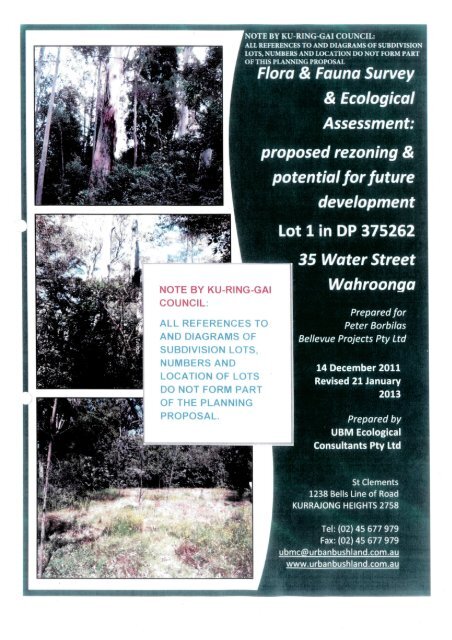The image appears to be a digitally created poster or page from a report, featuring a mix of photographs and text. On the left side of the poster, there are three vertically aligned photos depicting wooded areas and open grass fields, all taken outdoors during the daytime. The top and middle images show dense woods with trees, while the bottom picture displays a cleared area with trees in the background. The photos are somewhat overexposed and predominantly feature dark green, black, brown, and beige colors.

The right side of the poster contains a substantial amount of text. At the top, in white print, the title reads, "Flora and Fauna Survey and Ecological Assessment, Proposed Rezoning and Potential for Future Development." Following this, it specifies "Lot 1 in DP 375262, 35 Water Street, Barunga." Further down, it mentions the preparation details: "Prepared for Peter Berbilius, Bellevue Projects Pty Ltd, 14 December 2011, revised 21 January 2013, prepared by UBM Ecological Consultants Pty Ltd," along with their addresses and phone numbers in smaller print.

A central white text box stands out with a note from the Cooringay Council, stating, "All references to and diagrams of subdivision lots, numbers, and location of lots do not form part of the planning proposal."

Overall, the poster combines real photos and detailed text to convey information about a land development project and ecological assessment.